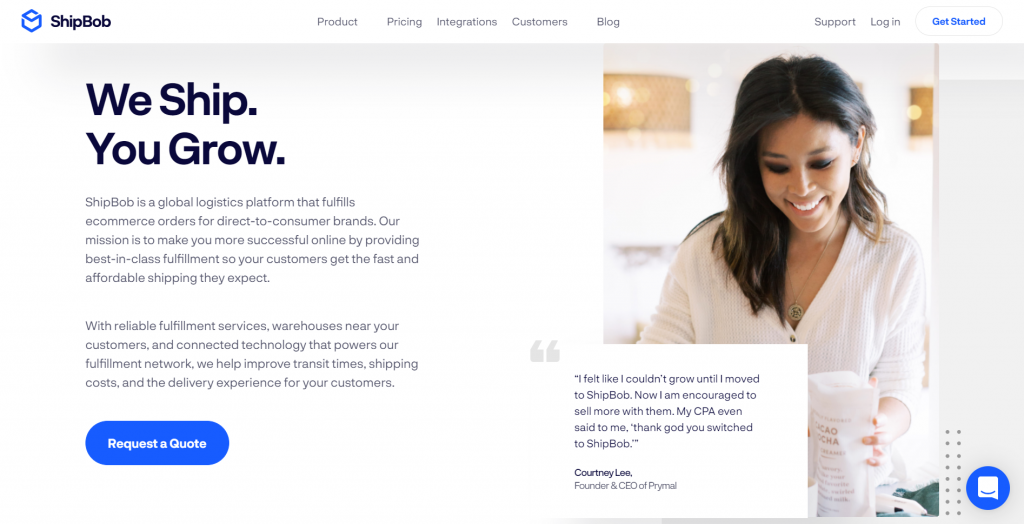In the top left-hand corner, there is a blue box symbol labeled "ShipBob." Across the top bar, the menu options read: Product, Pricing, Integrations, Customers, Blog, Support, Login, and a blue "Get Started" button. Below this menu, there is a boxed text that reads: "We Ship, You Grow. ShipBob is a global logistics platform that fulfills e-commerce orders for direct-to-consumer brands. Our mission is to make you more successful online by providing warehouses near your customers and connected technology. We help improve transit times, shipping costs, and the delivery experience for your customers." A blue button with white text says "Request a Quote."

To the right, there is a picture of a woman packaging a product, looking down and smiling. Below this image, a boxed quote reads: "I felt like I couldn't grow until I moved to ShipBob. Now I'm encouraged to sell more. My CPA even said to me, 'Thank God you switched to ShipBob.'" The quote is attributed to Courtney Lee, though the rest of her title is slightly blurred.

In the bottom right-hand corner, there is a blue circle with a white chat bubble icon, indicating a chat feature.